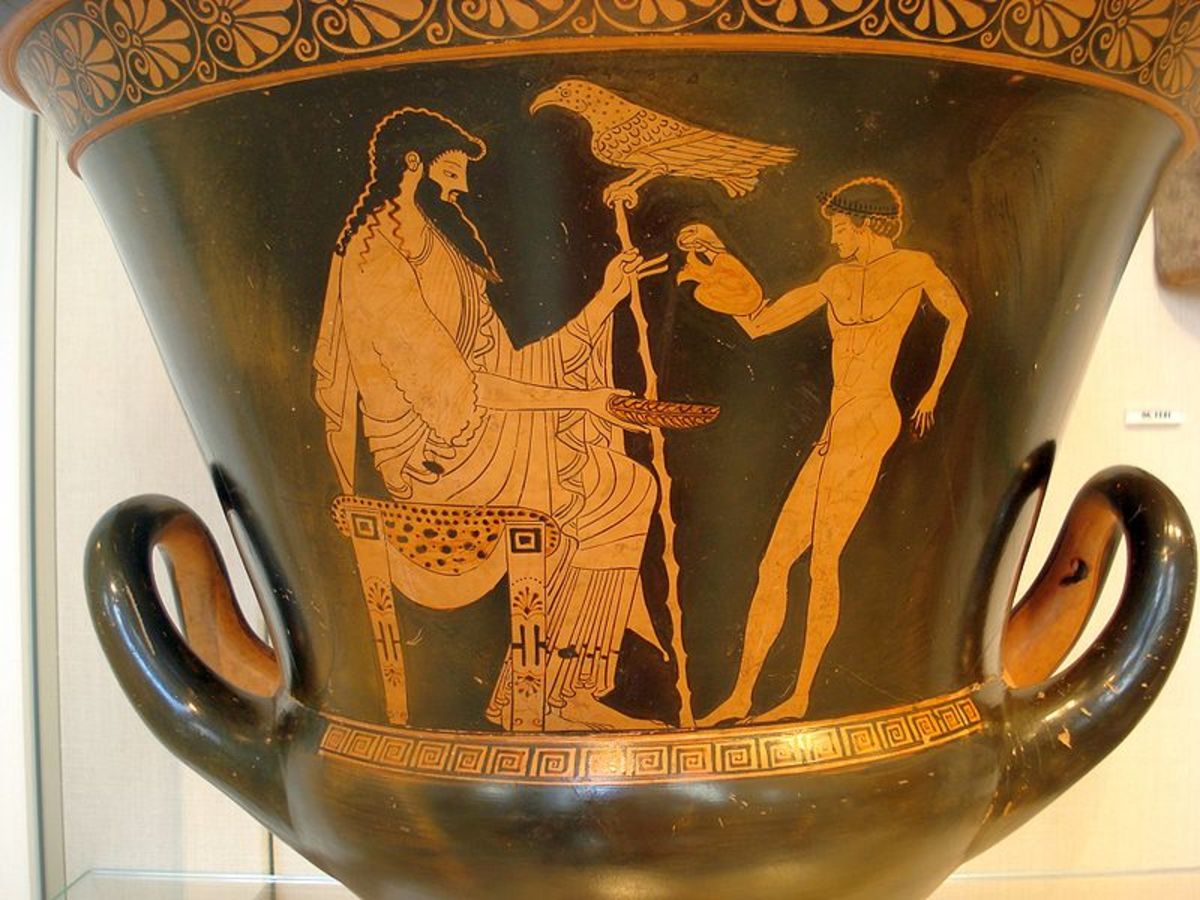This close-up photograph depicts a large, likely Greek vase, characterized by its distinct black and gold colors. The vase, which features two small upward-curving handles, exhibits a shape that narrows at the bottom and broadens towards the top. Detailed golden illustrations adorn its surface. Central to the decoration is an image of a seated bearded man with long hair, dressed in a robe, holding a staff with a bird—likely a raven or hawk—perched on top. The man extends a container towards a naked, young man standing before him, adorned only with a laurel around his head. This young man is depicted pouring liquid from a vessel into the container held by the older man. The presence of a small sign in the background suggests that the vase is displayed in a museum.